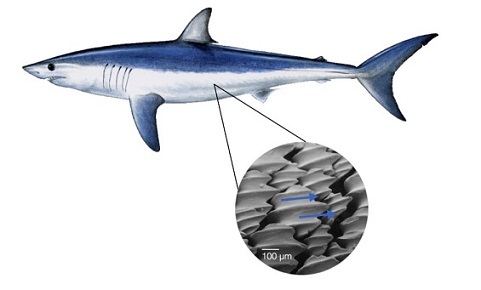This detailed illustration depicts a shark with a primarily blue top half and a white or light silver underside, possibly resembling a mako or blue shark but with generic features. The shark, positioned against a plain white background and facing left, showcases a mixture of colors: its body and side fins are blue, while the top of its dorsal fin is gray. The tail, which is also blue, has a longer upper lobe compared to the lower one. Notable features include a pointed nose, a large black eye, and five visible gill slits. The shark spans about three inches from the tip of its nose to the tail.

Inside the diagram, a zoomed-in circular thumbnail originating from the belly area provides a microscopic view of the shark’s skin texture. This close-up reveals grey, overlapping scales or shells with raised and pointed edges, indicating the rough texture of the skin. The thumbnail includes two blue arrows pointing left to right, indicating some detail about the skin structure. Beneath this inset is text stating "100 micrometers," reinforcing the microscopic scale of this detailed view. The intricate illustration combines various anatomical and microscopic details to provide a comprehensive representation of the shark.